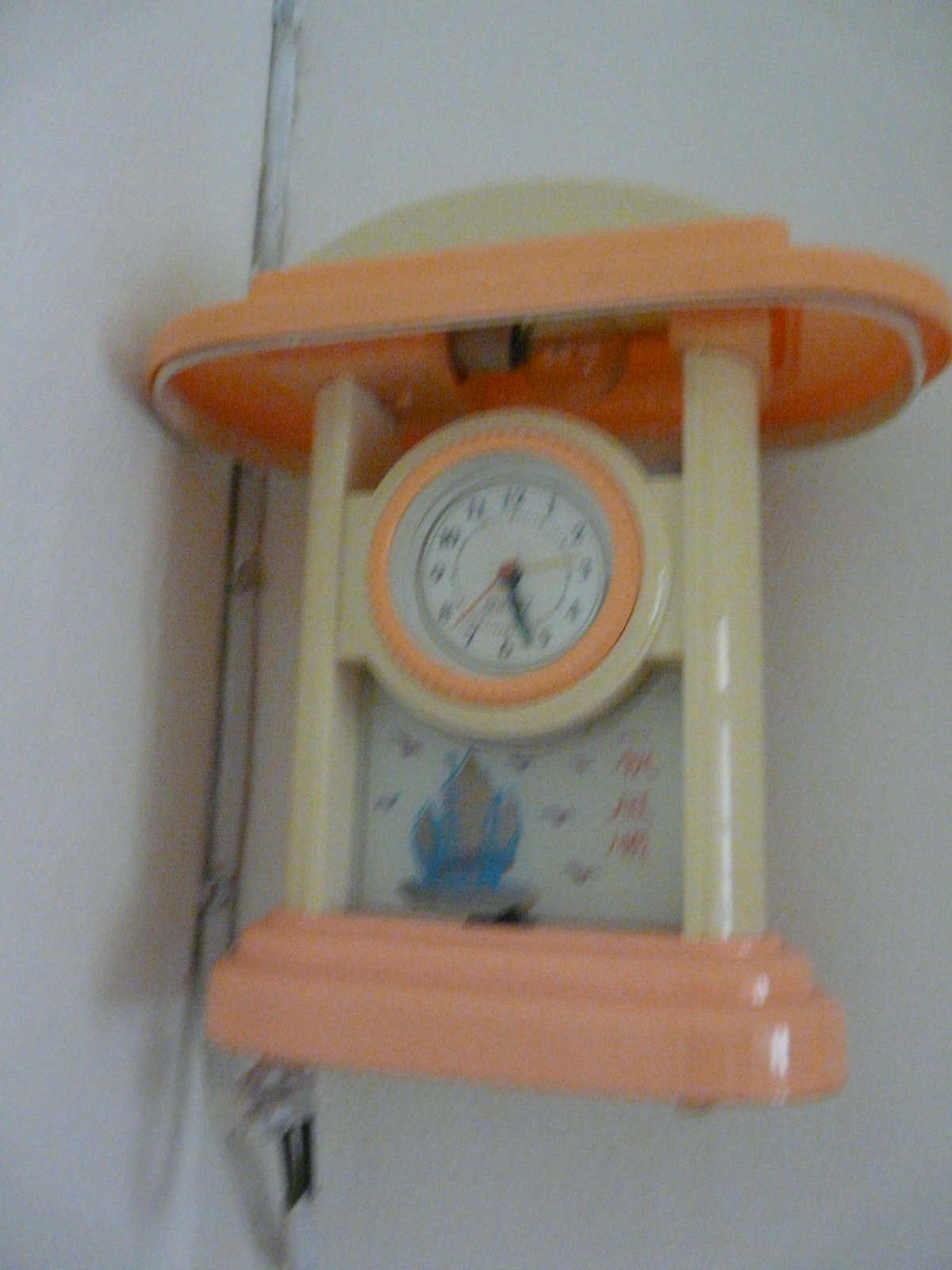The photograph is a blurry, color image showcasing a toy clock mounted on a white wall, particularly in a corner. The toy clock features a whimsical design, resembling a doll-like structure. It is composed of soft, pastel-like colors: prominently light orange and very light off-white, almost yellow. The clock face is traditional, circular, and white with black numbers, black hour and minute hands, and a red second hand. Surrounding the clock face is an orange circular frame.

The clock structure includes a white plastic dome at the top, bordered by an orange arc. Two white pillars extend from this dome, connecting to an orange base at the bottom. This base, together with the dome, forms the structural support, reminiscent of palisades. 

An unlit light bulb is screwed into the top of the frame, suggesting the clock might light up. Below the clock face, there’s a graphic element in blue, although the details are unclear due to the photograph’s blurriness. The playful blend of colors and the addition of unique elements like the light bulb reinforce the impression of the clock being both functional and decorative.